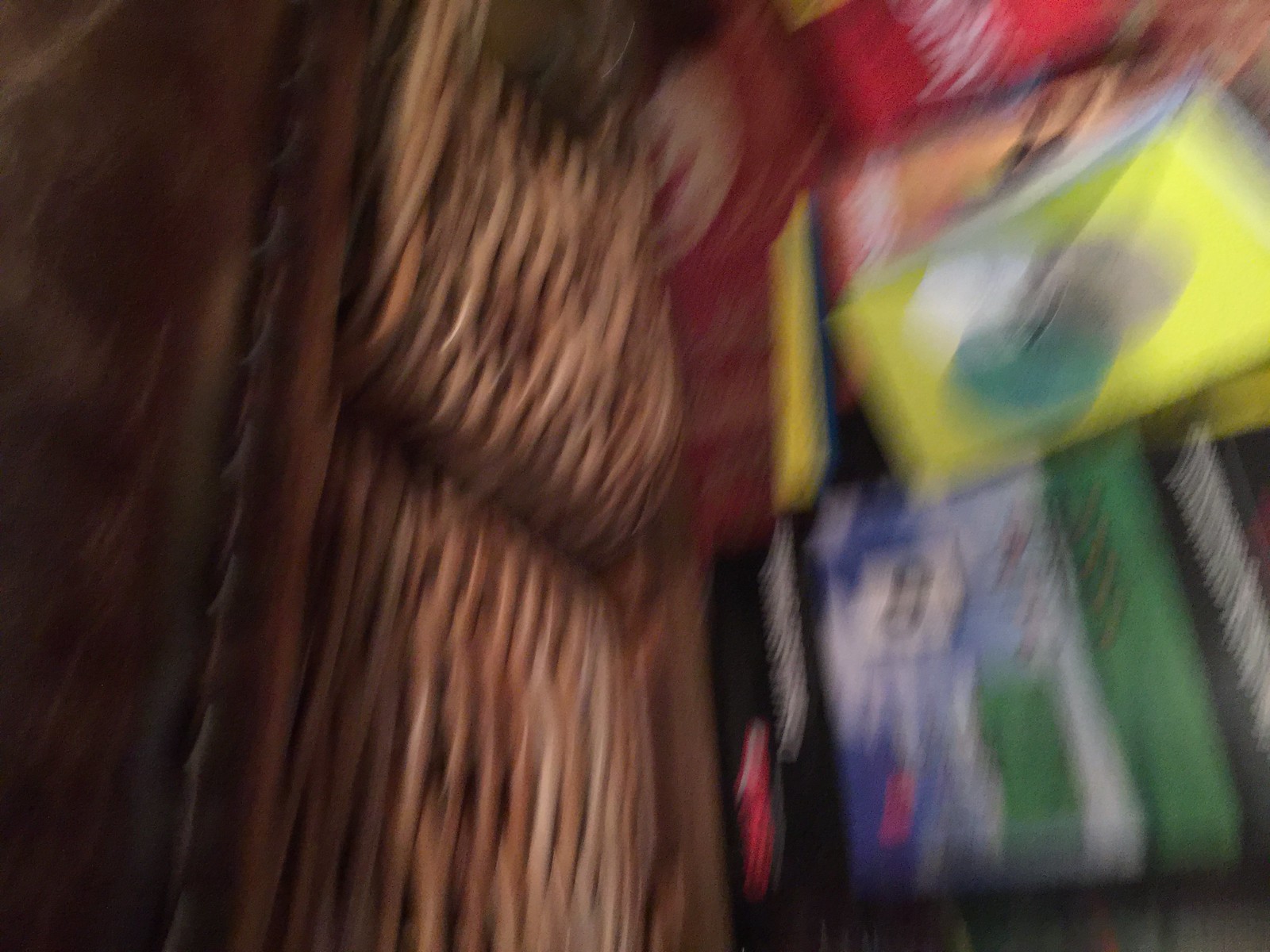This is a very blurry image taken at an angle, depicting a cluttered scene that is difficult to decipher clearly. On the right side, it appears there are several packages and books, including a notable large yellow book cover with blue, white, and gray colors, and a thick rectangular book featuring a skyscape with a green border at the top. On the left side of the image, there seems to be a brown and tan couch or possibly a leather trunk containing multiple folded items. Scattered among the contents, various items with different colored packaging can be found, including yellow, blue, red, orange, and green, possibly chair covers. The background contains some indistinct black and white shadows, adding to the overall blur of the photo.